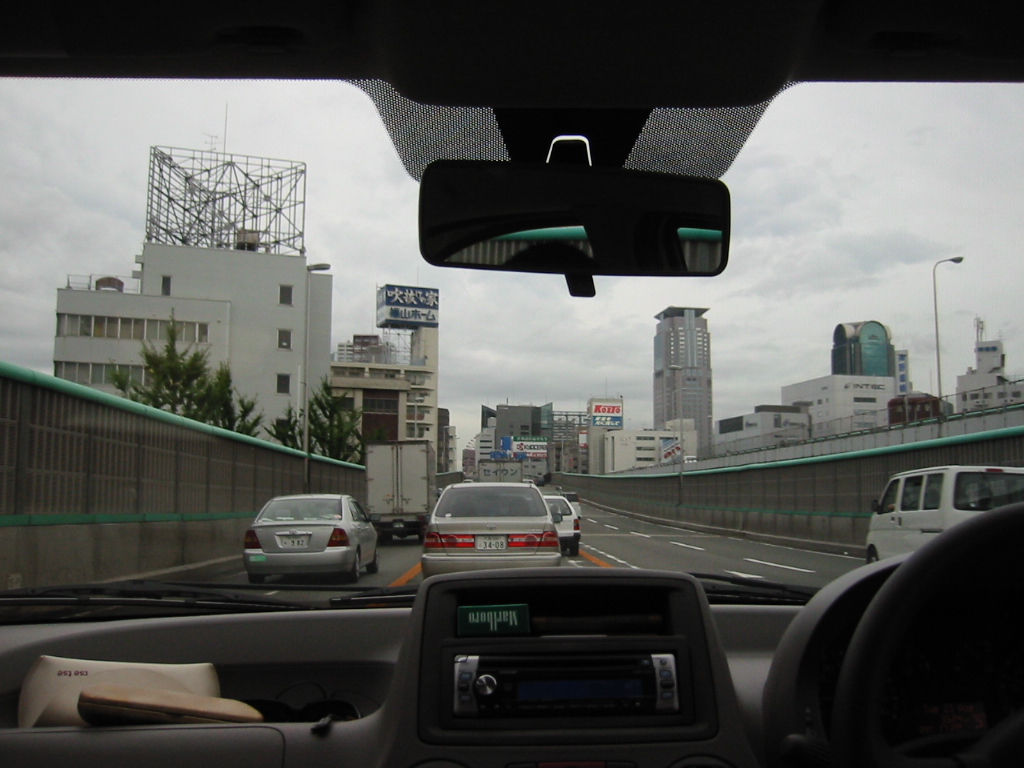A photo taken from inside a car captures the experience of driving into a bustling city. The interior of the car reveals the dashboard with a radio and, just above it, a slot holding a green pack of Marlboro menthol cigarettes. To the left of the radio, another slot contains what appears to be some books. The scene outside the windshield shows a stretch of traffic with a gray car directly ahead, followed by a white car, and another gray car to the left with a semi-truck positioned ahead of it. A concrete barrier topped with a green fence divides the lanes of traffic. Dominating the left side of the frame is a tall, white building crowned with a radio antenna tower. In the background, a building with Japanese writing on it adds to the urban scenery.